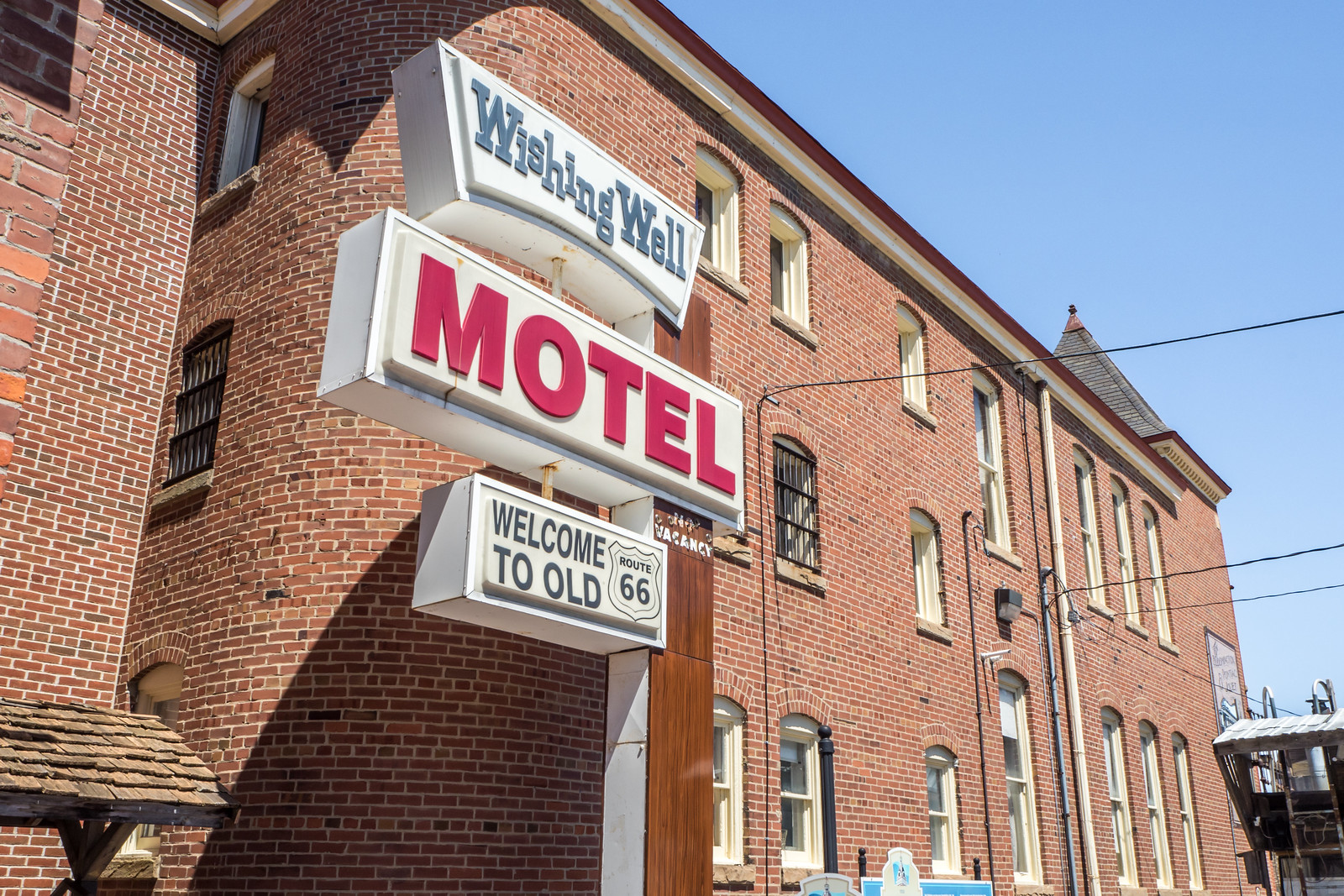The image depicts an old, three-story brick building with a rich reddish hue, viewed from the front left side. The structure curves along one edge, almost giving it a tower-like appearance, and features numerous windows with white panes, some of which are barred on the second floor. Against the backdrop of a clear blue sky, a network of telephone or communication wires connects to the building. On the lower left side of the picture, there is a white sign on a wooden pole. At the top of the sign, in blue lettering, it reads "Wishing Well." Below that, in large red letters, it says "Motel," and further down, in blue text, it reads "Welcome to Old Route 66," next to a symbol resembling a Route 66 badge. A small thatched covering, possibly the top of a wishing well, is also visible in the bottom left corner. Additionally, a long white water spout can be seen halfway down the building. The overall scene is nostalgic, evoking a sense of historical charm.